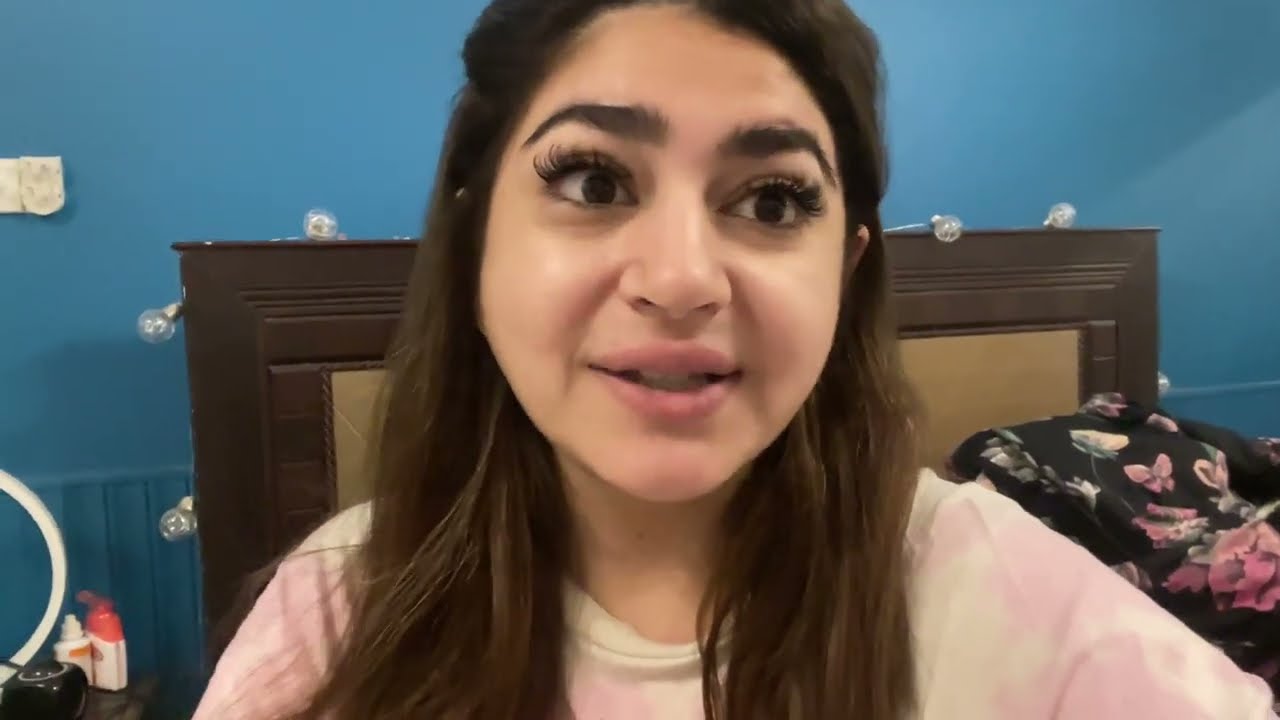The image captures a close-up shot of a young woman in her late teens or early twenties, centered against a bedroom backdrop. She has long, dark brown hair cascading past her shoulders and is wearing a pink and white tie-dye shirt. Her face, with thick eyebrows and long eyelashes, hints at the use of makeup, possibly including fake lashes. Her gaze is directed slightly to the right, with her lips subtly parted.

The room behind her features a wooden headboard with tan upholstery, against a blue drywall. The headboard is adorned with large lightbulbs strung together along its frame. Over her left shoulder, a black floral-patterned blanket, decorated with pink flowers, is visible. Additional details in the background include a potential dresser and bottles, possibly medicine, near what looks like a ring light, suggesting she might be setting up for a selfie or a podcast recording.